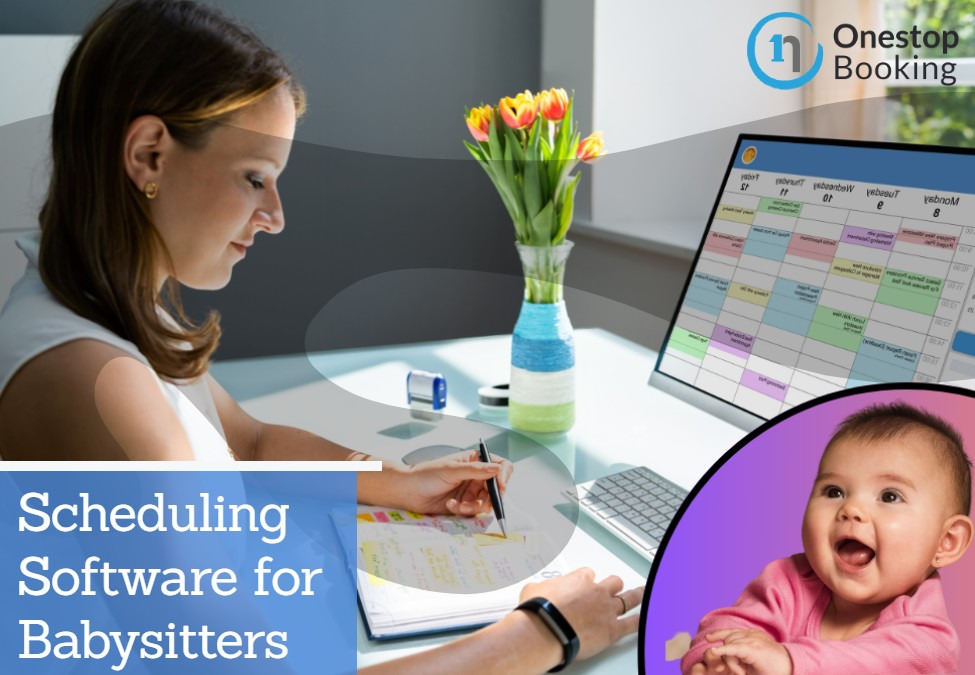The image is an advertisement for babysitting services featuring a woman seated at her desk. To the left, the side view shows her with shoulder-length, dark brown hair neatly tucked behind her ears. She is dressed in a sleeveless white shirt and is smiling softly as she reviews her calendar on both a notebook and a desktop computer in front of her. Her left hand, adorned with a smartwatch and gold earrings, holds a pen poised over the paper, while her right hand steadies the page. Positioned to the left of the woman, a vibrant vase filled with red and yellow tulip flowers and abundant green leaves adds a pop of color to the scene. The vase features a gradient of light blue, dark blue, white, and green bands from top to bottom. The desktop shows a scheduling software interface, with a visible keyboard and a computer screen displaying the calendar she is concentrating on.

In the top right corner, black lettering reads "One-Stop Booking" next to a blue and black stylized 'N' symbol. The bottom left corner features a blue box with white lettering stating "Scheduling software for babysitters," emphasizing the ad's purpose. Within the lower right corner, a pink and purple half-circle frame contains an image of a baby girl wearing a pink onesie, her head slightly tilted up in a wide, cheerful smile. The scene effectively conveys a professional yet personable environment, highlighting software aimed at assisting babysitters with their scheduling needs.